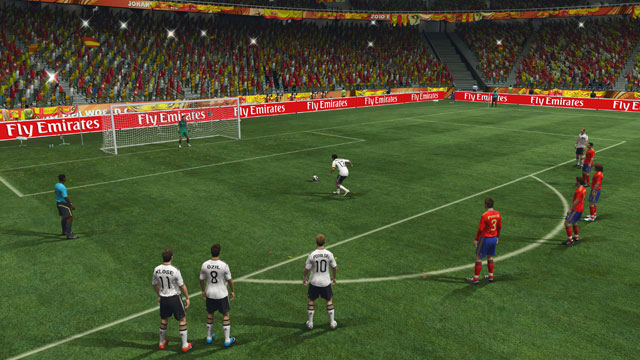In this rectangular digital image, we see a vividly rendered scene from a video game that replicates a high-stakes soccer match. The foreground features a vast expanse of lush green, artificial turf. Arrayed in a semi-circle and facing away from us are several intricately designed soccer players, each in mid-action, eagerly watching a critical moment unfold. The two opposing teams are distinctly attired; the players on the lower left are dressed in white shirts paired with black shorts, while the players on the right sport blue shorts and vibrant orange long-sleeved tops. 

Our attention is drawn to a pivotal player from the team in white and black, who is poised to take a crucial shot towards the goal. The goal itself is guarded by a player in a striking all-green outfit, emphasizing his role as the goalkeeper. Adding to the realism, an umpire is positioned on the lower left, overseeing the play. 

In the background, pixelated stands are teeming with a virtual crowd, reduced to colorful splotches that suggest a dynamic audience. Among the crowd, arrays of lights—likely spotlights—shine outward, enhancing the game's immersive atmosphere. Adding a touch of authenticity, the perimeter of the stands is adorned with virtual signage displaying the slogan, "Fly Emirates!" The overall scene captures the intensity and excitement of a live soccer match, brought to life through stunning digital artistry.